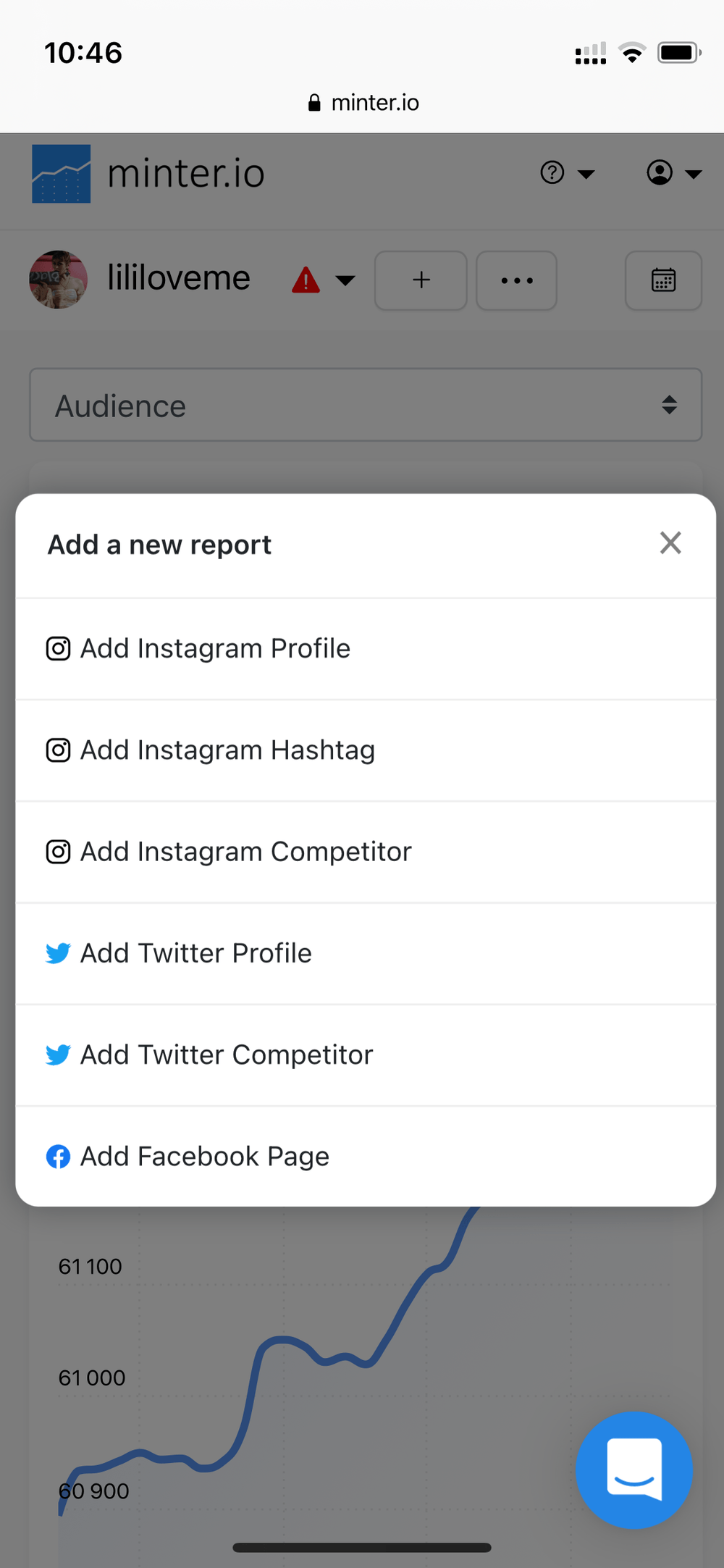In the image, we see a phone screen with a light background. At the top left corner, the time is displayed as 10:46. To the right of the time, standard icons for Wi-Fi, signal strength, and battery status are seen. In the center of the top bar, there is a small black lock icon and the text "mentor.io".

The screen background appears grayed out, but it's possible to make out an avatar combined with the "mentor.io" logo. To the right of the logo, there are three icons – a question mark, a person, and a down arrow.

Below this section is a username "lililoveme" accompanied by a somewhat indistinct profile picture that appears pink and features a person in the center. Adjacent to the username is a red warning triangle with an exclamation mark in it. This area also contains a drop-down marker, a plus button, an ellipsis button, and a calendar button.

Following this, we find an audience drop-down option. At the bottom of the screen is a graph featuring a blue line trending upward along with unclear Y-axis labels that alternate numbers such as 61, 100, 60, and 900.

The central feature of the image is a prominently highlighted box with the text "Add New Report." Below this, several options to add various social media profiles and competitors are listed. These options are labeled:

- Add Instagram Profile (with Instagram logo)
- Add Instagram Hashtag (with Instagram logo)
- Add Instagram Competitor (with Instagram logo)
- Add Twitter Profile (with Twitter logo)
- Add Twitter Competitor (with Twitter logo)
- Add Facebook Page (with Facebook logo)

In the bottom right corner, there is a blue circle featuring a white bookmark icon in the center, which surprisingly has a smiley face on it.